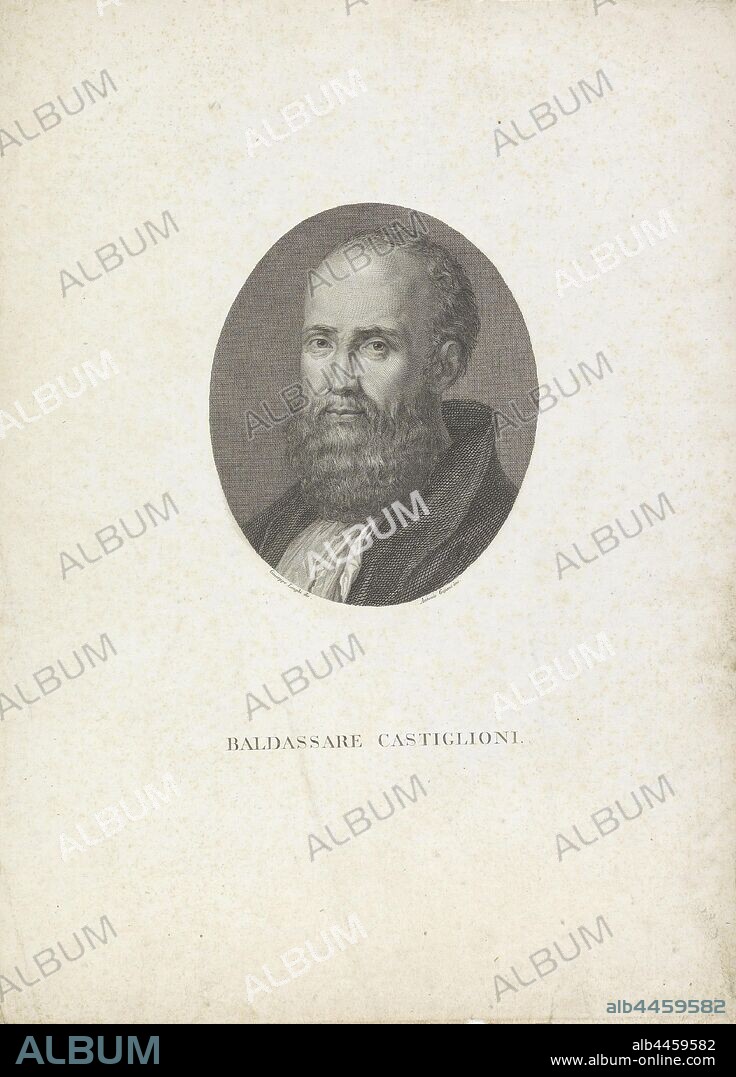The image depicts an antiquated-looking album cover featuring a weathered, slightly creased piece of paper with a tan, darkish white background. The surface is adorned with the word "album" in a diagonal slant, alternating between black and white text. Central to the design is a detailed black and white pencil illustration of a stern-faced, balding man with a large beard, wearing a dark coat with a white kerchief. The illustration exudes a hand-drawn quality reminiscent of antique currency portraits. Beneath the portrait, the name "Baldessare Castiglione" is inscribed in black type. The bottom of the image has a distinct black footer rectangle. On the lower left within this footer, "album" is written in blue text, while on the lower right, the code "ALB4459582" appears in white text, with the same code in light blue directly above it against the tan backdrop. Also, the URL "www.album-online.com" is displayed beneath the code in the black section, suggesting a modern reproduction or reprint service for this classical album cover.